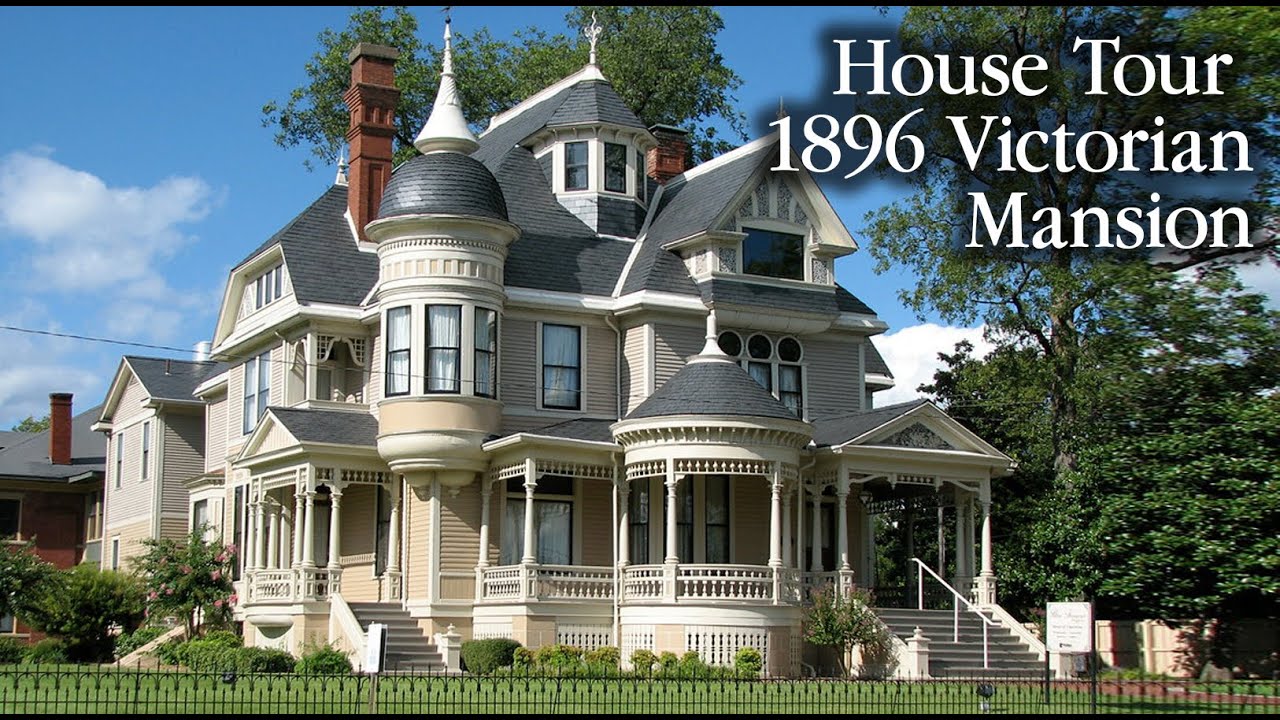This photograph features a beautifully preserved 1896 Victorian mansion under a clear blue sky, destined for a blog post or YouTube video as indicated by the bold white text “House Tour 1896 Victorian Mansion” in the upper right corner. The three-story mansion stands proudly at the center, boasting a cohesive yet unique architecture with sloped, rounded, and pointed roofs, including dome-shaped turrets topped with white spires and large, prominent windows. The facade is cream-colored with white pillars, detailing around the windows, and the rooftops, capped in gray, contributing to its charming aesthetic. 

In the foreground, a well-manicured bright green lawn bordered by a short black wrought iron fence with pointy tops stretches across the bottom of the image. To the right, a red brick pathway angles towards the house, leading to concrete steps that ascend to a half-circle porch, reminiscent of a gazebo, then continuing up to a turret on the second floor. There's also a covered porch accessible via stairs on the right-hand side. A large tree with vivid green leaves partially frames the scene, while smaller bushes nestle alongside the left side of the house. Notably, two brick chimneys rise from different sections on the roof. In the distance on the left, just barely in frame, is a glimpse of a red brick house.